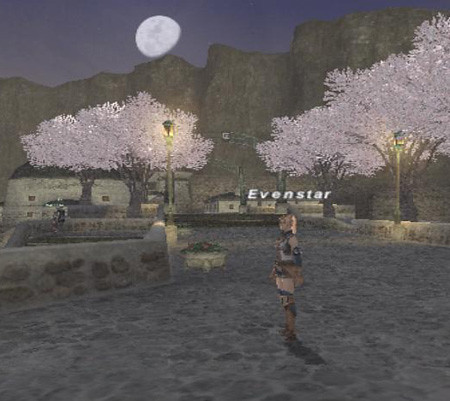In the pixelated nighttime image reminiscent of a video game, a female character with blonde hair, dark shorts, brown boots, and knee pads stands prominently. She appears to be holding a gun and is positioned on a grey stone walkway adorned with scattered gravel or pebbles. The character faces a grey wall embedded with rocks, while above her, a sign reads "Evenstar," suggesting the presence of a building, possibly a hotel, in the background. The scene is beautifully illuminated by a three-quarter moon hanging above sheer rocky cliffs. Striking white-leaved trees, possibly cherry blossoms, frame the image, their dark trunks contrasting vividly against the night. Two streetlights, with yellow glowing lamps, add a subtle, eerie ambiance to the scene, enhancing the pixelated yet enchanting atmosphere.